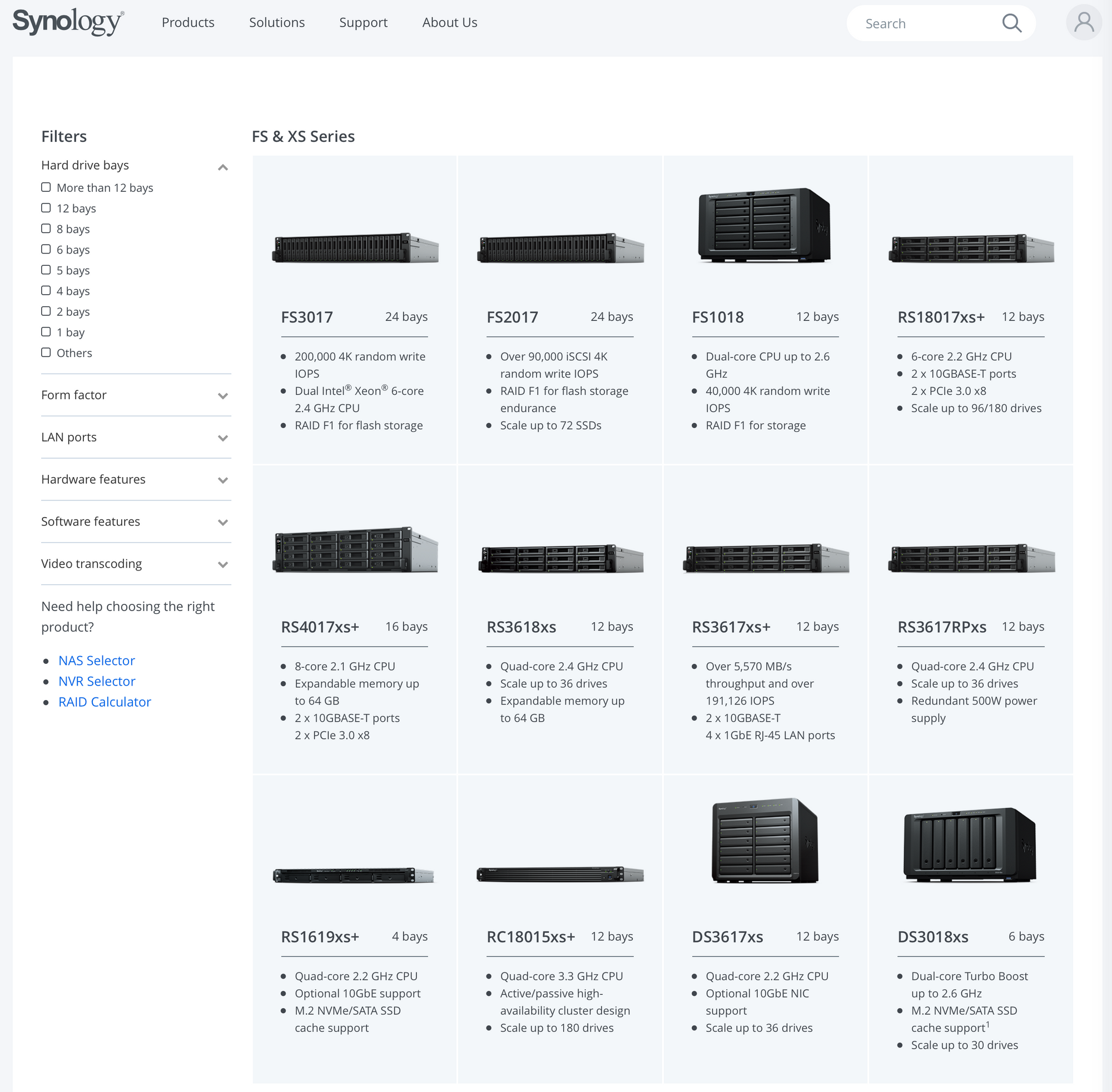The image is a screenshot from the Synology website, clearly indicated by the prominently displayed brand name at the top, spelled out as "SYNOLOGY." On the right side of the header, there are navigation tabs labeled "Products," "Solutions," "Support," and "About Us," followed by a search bar with an embedded search button and a user icon in the upper right corner for account access.

Descending from the "Synology" logo down the left-hand side, a white sidebar lists various filtering options beginning with "Filters" and "Hard Drive Bays." Below this, there are sections categorized by the amount of bays. Further filtering tabs include "Form Factor," "LAN Ports," "Hardware Features," "Software Features," and "Video Transcoding."

Towards the bottom of the sidebar, helpful tools are listed, such as "Need help choosing the right product," "NAS Selector," "NVR Selector," and "RAID Calculator."

In the main content area, central to the right of the sidebar, is a highlighted section for the "FS and XS Series," featuring images of various storage devices designed for corporate and server use. This section showcases three rows of four products each, neatly arranged and displayed to inform prospective buyers. The overall design is functional and aimed at assisting users in navigating through the various product offerings efficiently.